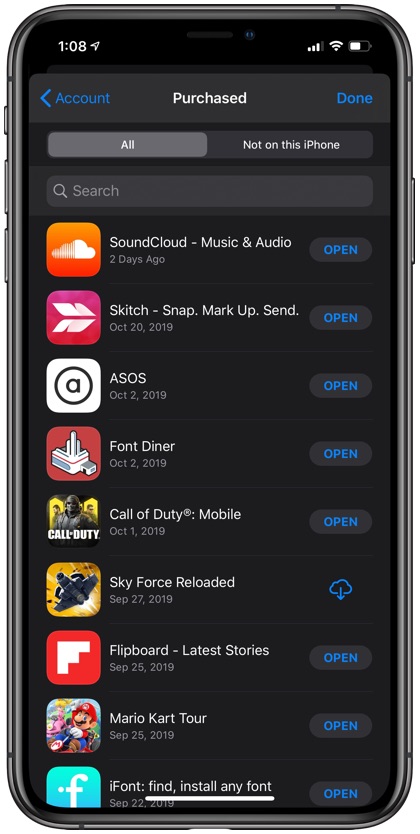The image depicts a mobile device featuring a predominantly black screen that displays a list of purchased applications. The apps are organized in a vertical sequence descending down the screen. Among the showcased apps are SoundCloud, Skitch, Font Diner, Call of Duty Mobile, Sky Force Reloaded, Flipboard, Mario Kart Tour, and iFont, among others. The screen also includes a search bar located at the top, likely intended for searching through the apps listed on this screen. The mobile device appears to be in an app management or purchase history section, allowing the user to view and access their recently acquired applications.